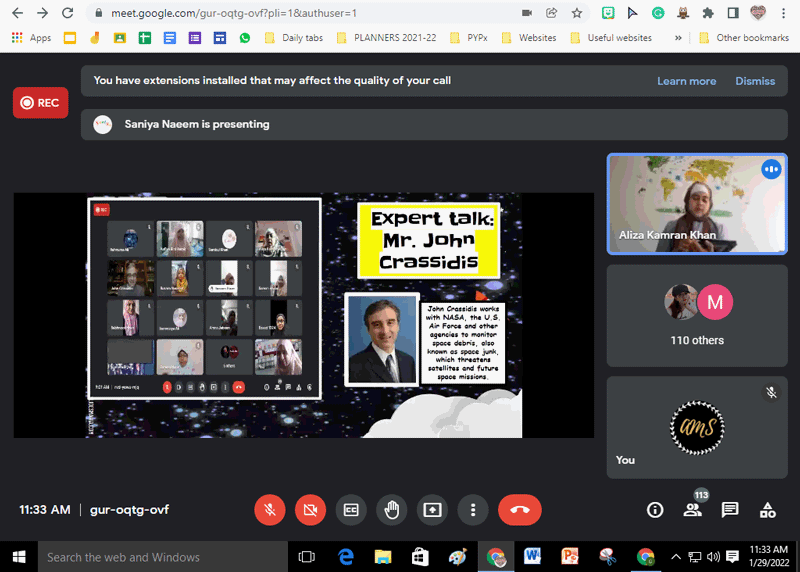The image is a detailed screenshot of a Google Meet session captured within a web browser. The URL is visible at the top, displaying "meet.google.com" followed by an assortment of letters and numbers. The browser background is a very dark gray, lending a focused and professional look to the screenshot.

At the top of the screen, a notification written in white font states, "You have extensions installed that may affect the quality of your call." This message is notable for ensuring users are aware of potential issues that might impact their conference experience.

In the upper left corner, a prominent red oblong box displays the word "REC" in white font, symbolizing that the meeting is being recorded. Adjacent to this box, there is a white circle, adding to the interface's recording indicators.

The main section of the screenshot features the typical layout of a Google Meet conference, showcasing a grid of squares. Each square contains the video feed of a participant, illustrating the collaborative nature of the meeting.

To the right of the participant grid, there is an oblong rectangular section with a white background. Displayed in black font are the words, "Expert Talk." Below this heading, the name "Mr. John C-R-A-S-S-I-D-I-S" is spelled out. Underneath the text is a professional headshot of Mr. John Crassidis, a white man in his mid-forties with dark brown hair. He is dressed in a gray suit, white shirt, and a silver-gray tie, exuding a professional demeanor suitable for the expert talk being presented.

Overall, this screenshot provides a comprehensive glimpse into a live Google Meet session, emphasizing the functional elements and the primary speaker's details.